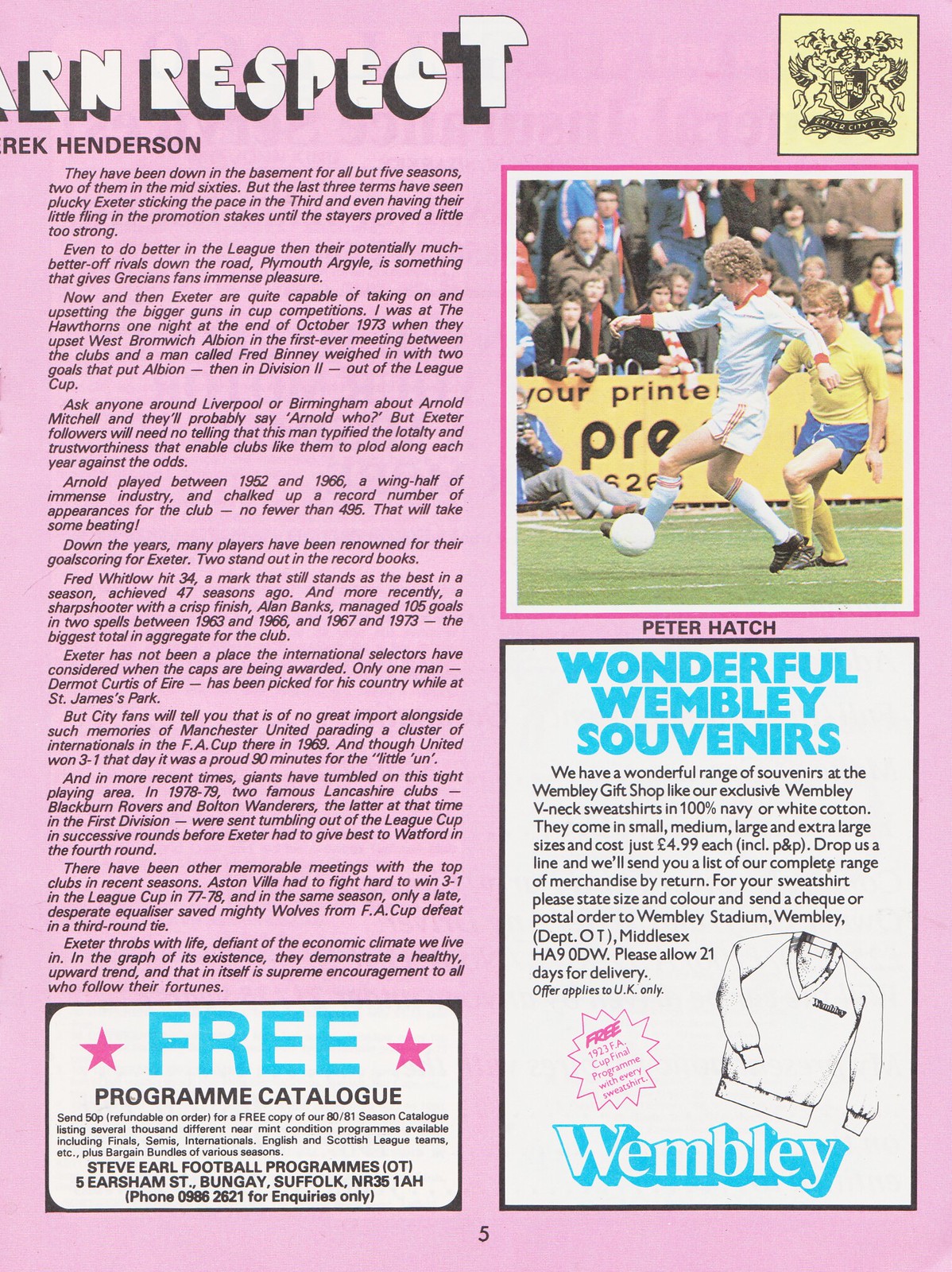The image is a scanned page from a soccer magazine, specifically page 5, featuring a prominent pink background split into two halves. On the left half, there's a featured article titled "Henderson," followed by an announcement of a free catalog for Steve Earl football programs. The right half showcases two main segments. 

At the top, there’s a partially obscured text reading "R-E-S-P-E-C-T," with the "T" slightly elevated, appearing in white text with a black shadow. Just below this, in the upper right corner, a yellow square with a black display is present, followed by a photograph of two soccer players in the midst of a game. One player, dressed in a white jersey with white shorts and black shoes, is poised to kick a white soccer ball. Behind him, another player wears a yellow shirt, blue shorts, and yellow socks. The caption below the photo reads "Peter Hatch."

Beneath the photograph, an advertisement for Wembley souvenirs features prominently. The ad highlights a collection available at the Wembley gift shop, including Wendy V-neck sweatshirts made of 100% navy or white cotton. It specifies that the sweatshirts are available in small, medium, and extra-large sizes for £4.99 each, including postage and packaging. It provides details for ordering and notes a 21-day delivery period. Illustrations include a black sketch of a long-sleeved sweatshirt and a pink star indicating "free inside," with the word "Wembley" in white text and a blue outline beneath.

The bottom right corner of the page contains another small square with the word "FREE" in blue text flanked by pink stars, coupled with the text "Program Catalog" and the number 5 centrally placed at the very bottom.